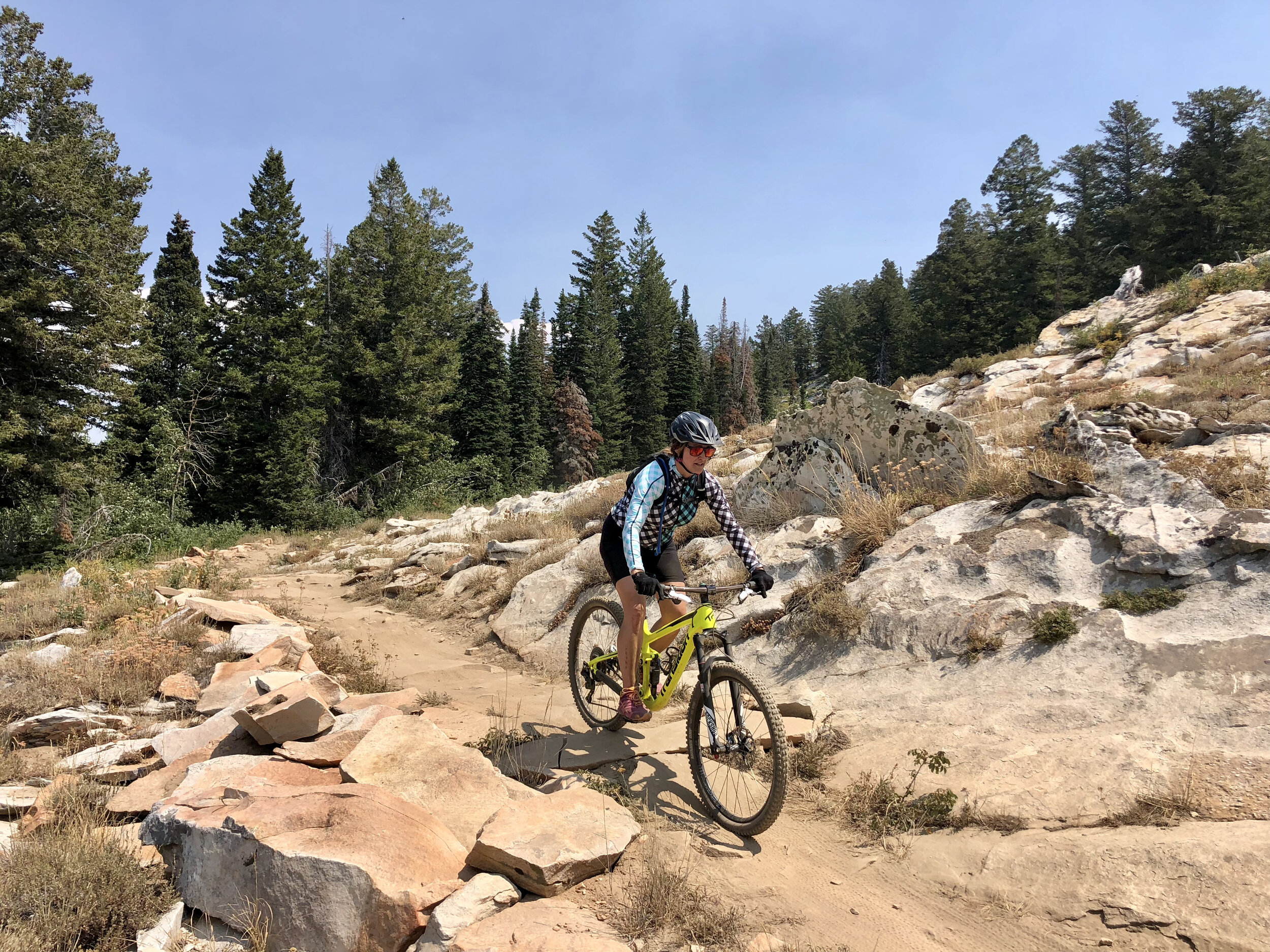In this outdoor photograph set in a rugged mountain terrain, a woman rides a bright yellow mountain bike along a narrow dirt path. She is equipped with a black and white helmet, red-tinted sunglasses, and long sleeves on a black and white polka-dot shirt with one blue sleeve. She also wears black biker shorts and distinct pink shoes. The trail she navigates is flanked by numerous large rocks and dry, brownish grass. Evergreen pine trees dominate the background, towering over the scene and giving the impression of a secluded, challenging environment. Small bushes are also visible to the left, further emphasizing the rough, rocky landscape through which she rides.